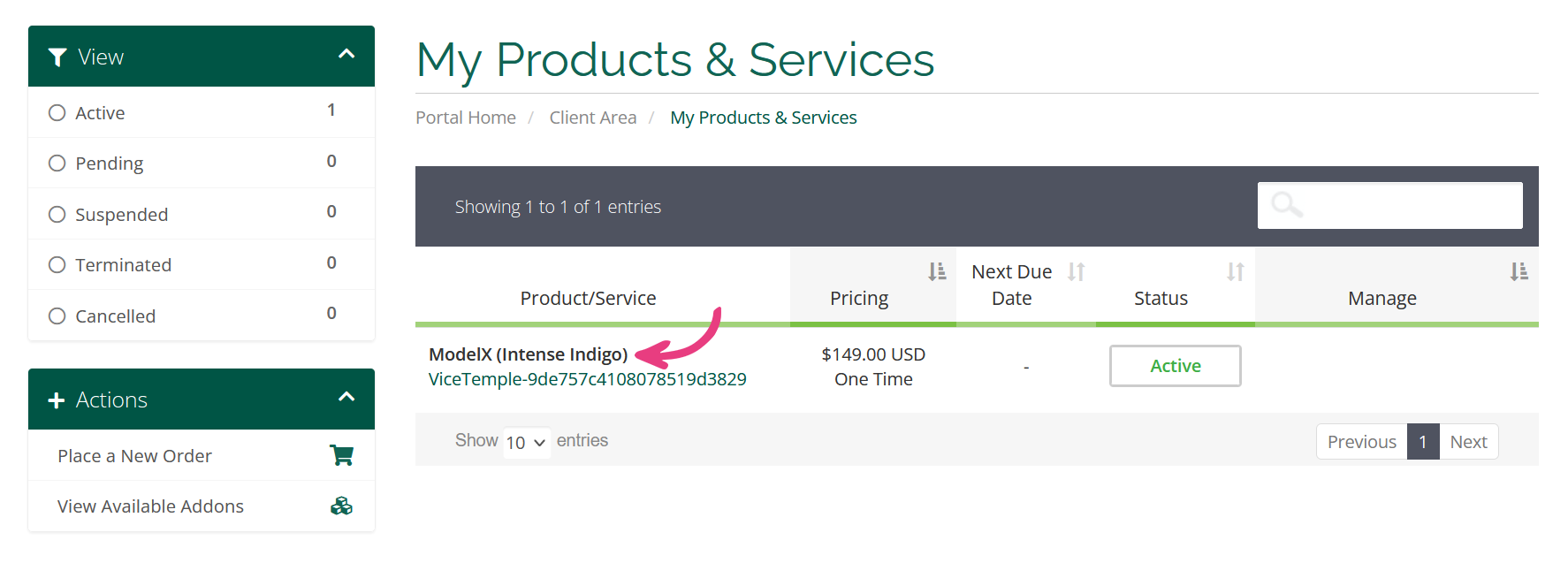This image shows a detailed view of a web portal interface, displayed in landscape orientation and divided into two main sections. The left section features a vertical menu with green headers, each functioning as expandable options.

The first header is a green rectangular box with the word "View" displayed in white font, accompanied by a filter icon and an upward caret symbol, indicating that it can be expanded or collapsed. Below this header, a list of filter options is visible, including "Active," "Pending," "Suspend," "Terminate," and "Cancel."

Beneath the filter section, another green box with white text reads "Actions," also featuring an up caret symbol. Under this header are two actionable options: "Place New Order" and "View Available Add-ons," each accompanied by relevant icons to their right.

The central section of the portal displays a white background, topped with a green header and thin underlining that reads "My Products and Services." Below the header, three options are visible: "Portal Home" and "Client Area" are in gray, while "My Products and Services" is highlighted in green, indicating the active section.

Directly below, a gray bar indicates that one entry is being shown with headers for a data table: "Product/Service," "Pricing," "Next Due Date," "Status," and "Manage." The first row under these headers lists a "Model X Intense Indigo" under the "Product/Service" column, marked by a red downward-pointing arrow. In the "Pricing" column, the cost is stated as "$149 US dollars." The "Next Due Date" field is blank. The "Status" column shows "Active" inside a gray box with green font, and the "Manage" column is currently empty.